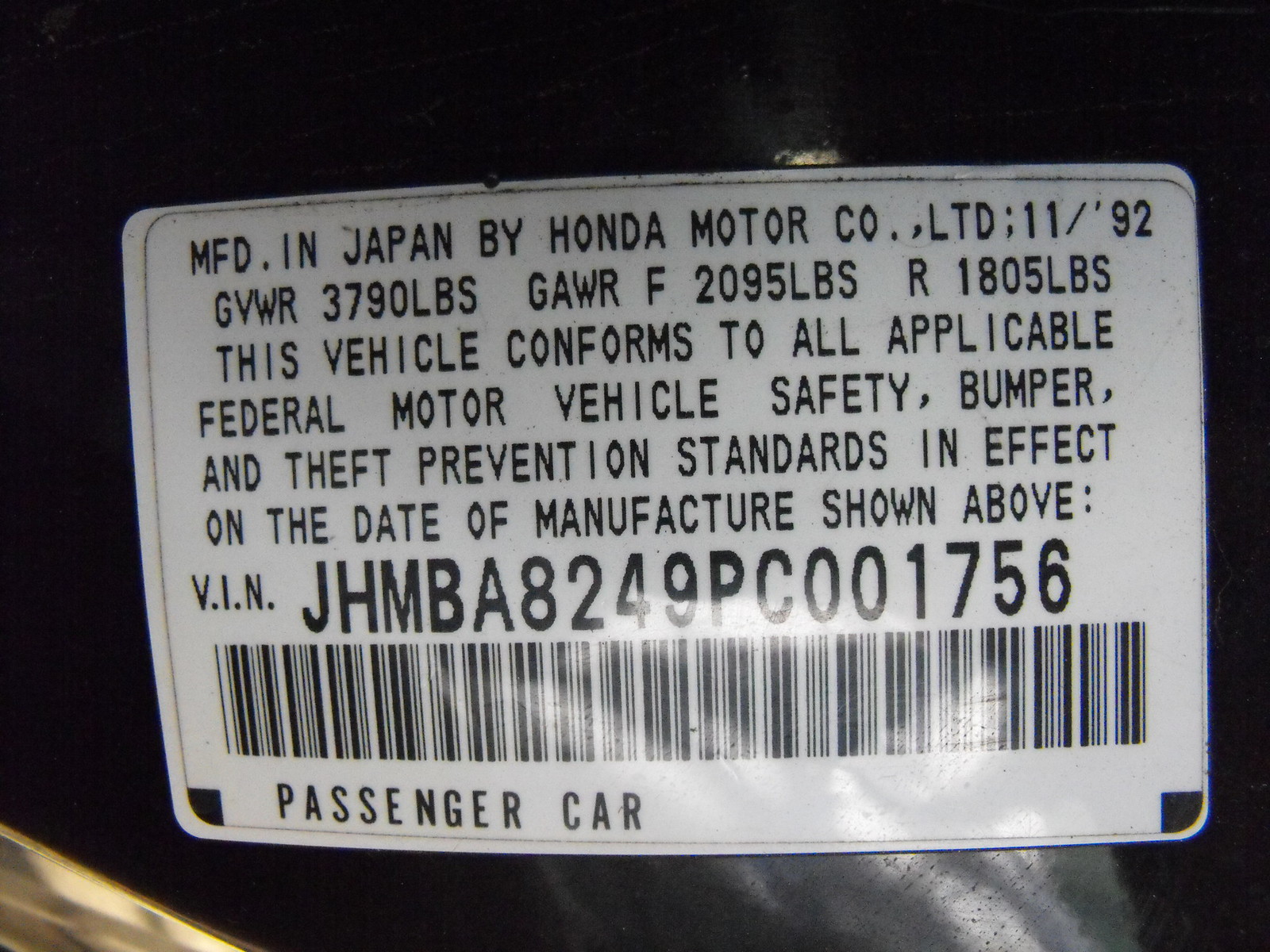The image shows a highly detailed, zoomed-in picture of a manufacturer's label affixed to a black metal surface of a Honda motor vehicle, possibly on its side. The prominent sticker, centrally positioned in the image, contains regulatory information. The text on the label states: "Manufactured in Japan by Honda Motor Company, LTD. 1192," indicating the year 1992. It specifies weight metrics such as GVWR 3790 lbs, GAWRF 2095 lbs, and GAWRR 1805 lbs. Additionally, the label confirms the vehicle's compliance with all applicable Federal Motor Vehicle Safety, Bumper, and Theft Prevention Standards effective on the date of manufacture. Below the compliance information, there's a VIN number, "JHMBA8249PC001756," followed by a barcode. The colors visible in the image are black, white, gold, and tan. The scene reflects light behind the camera, and the context suggests the photo was taken in an undefined indoor or outdoor setting, focusing purely on the label's details against the car's surface.